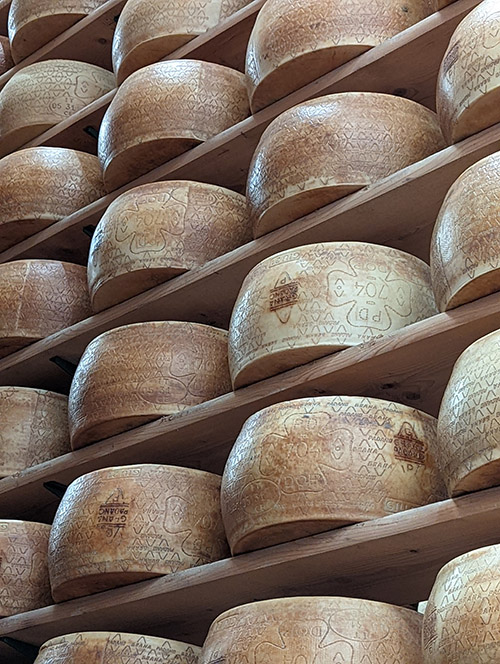The image depicts a set of round, antique-style containers, potentially wooden bowls or pots, displayed on a series of seven wooden shelves. Each container is adorned with intricate designs, including a motif resembling a four-sided clover or shamrock. Inscriptions such as "PD704" and "PDI704" are visible, alongside diamond-shaped patterns. The containers appear to be brown and light beige, giving them an aged, somewhat dirty or rusted look. Some containers feature a wood-burnt section with unreadable text in a square section, and bases with an indent marked "CIL." The overall setting resembles a storage or display setup, possibly indicating the items are stored or awaiting sale.